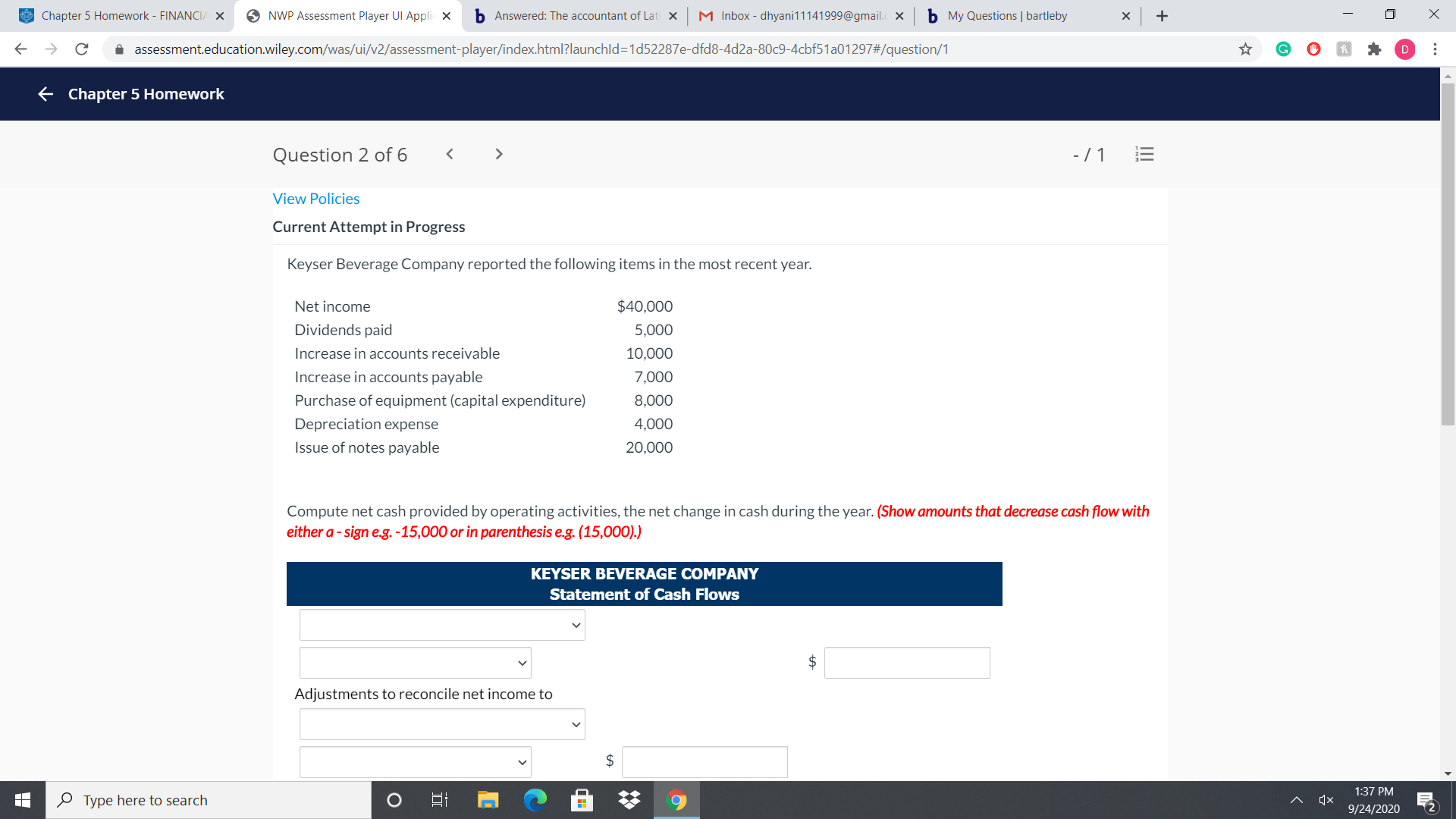This is a screenshot of a Chrome browser window with five open tabs. The tabs from left to right are labeled: "Chapter 5 Homework Finance," "NWP Assessment Player UI" (the active tab), "Answered: The Accountant of LA" on Bing, "Inbox" on Gmail, and "My Questions" on Bing. The URL in the address bar reads: "assessment.education.wiley.com/was/ul/v2/assessment-player/index.html?launchchild." Below the address bar, there's a navy blue header with white text displaying "Chapter 5 Homework" and a leftward-pointing white arrow. Beneath this header, the page shows the text "Question 2 of 6."